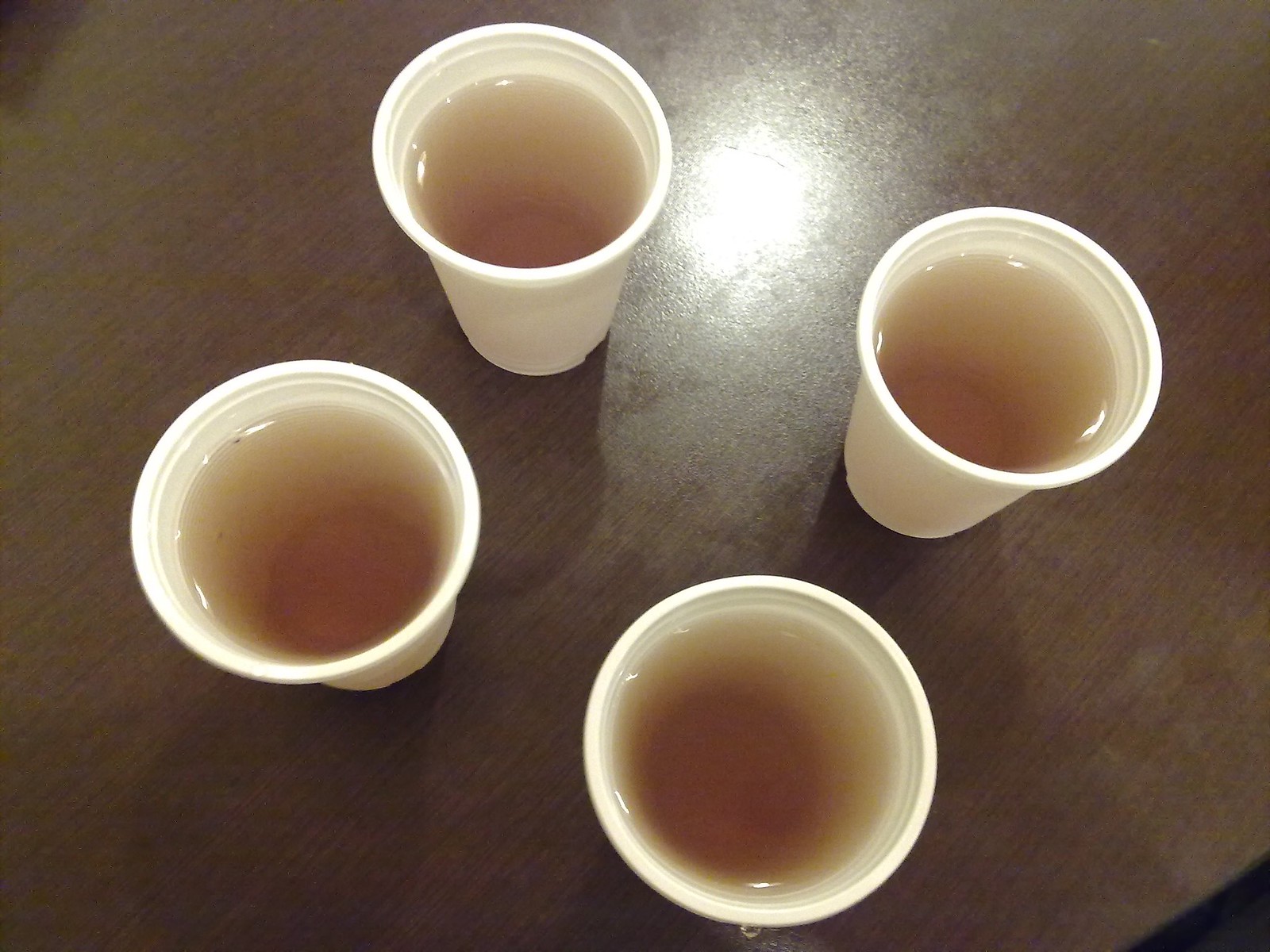This photograph, taken from above, captures a tabletop scene featuring four off-white plastic cups arranged in two rows of two, forming a square. Each cup is filled nearly to the rim with a light brown liquid, which appears to be a watery tea. The surface of the liquid is relatively clear at the top, gradually darkening as you look deeper into the cups. The light brown tabletop, which resembles faux wood grain and may be round, features a prominent reflection of an overhead light in the upper middle portion of the frame, creating a bright glare. The consistency in the liquid levels and the positioning of the cups highlights the symmetry of the arrangement against the plain but textured background.